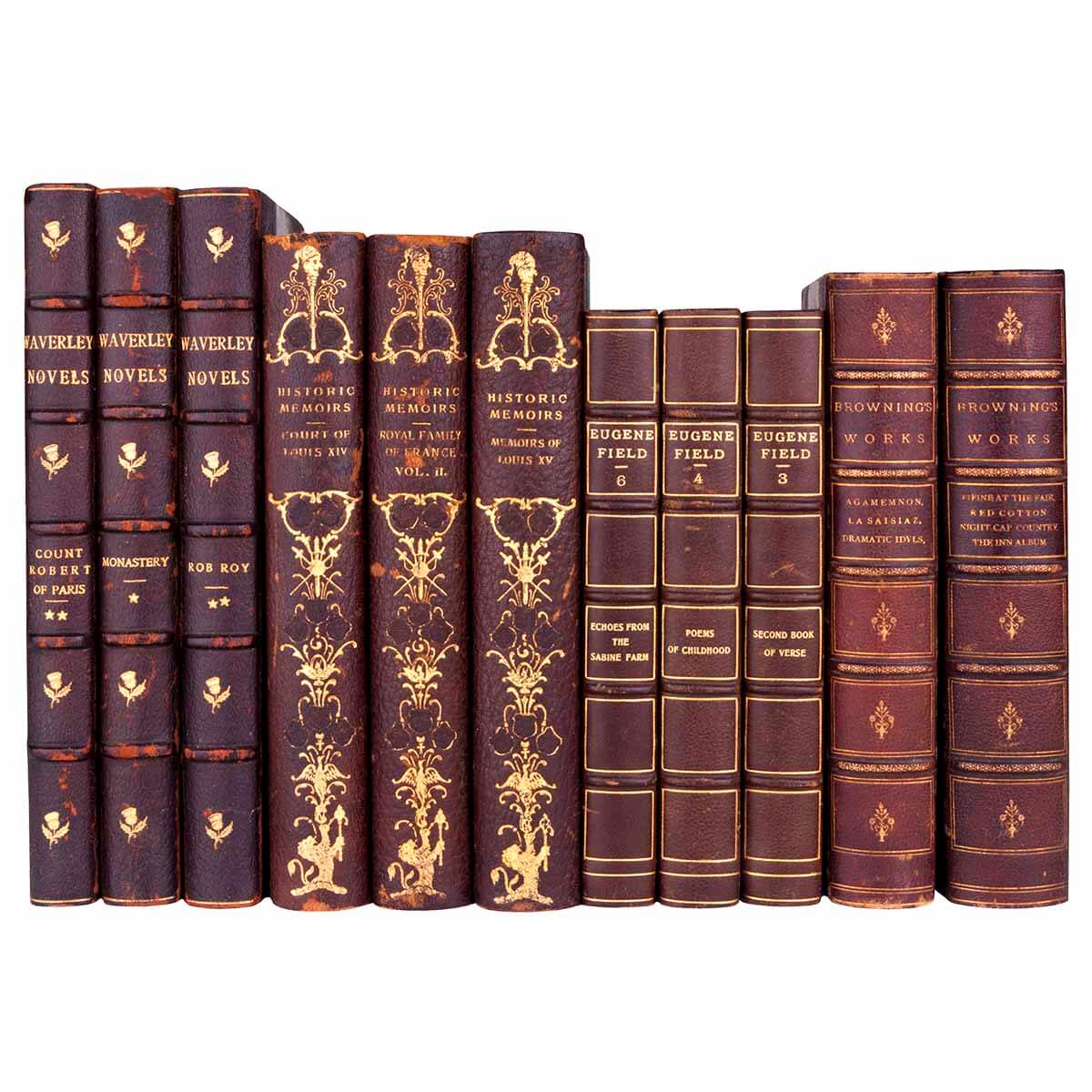The image features an arrangement of 11 leather-bound books with ornate gold leaf accents, laid out against a white background to mimic their appearance on a shelf. The books are a common burgundy color with gold text and illustrations on their spines, and can be separated into four distinct sets based on their titles and heights. The first three books on the left belong to the Waverly Novels series, with titles including "Count Robert of Paris," "The Monastery," and "Rob Roy." Next are three slightly shorter volumes from the Historic Memoirs series, titled "Court of Louis XIV," "Royal Family of France Volume 2," and "Memoirs of Someone XV," though the last title is not fully legible. The following trio of books bears the name Eugene Field, with titles like "Echoes from the Sabin Farm," "Poems of Childhood," and "Second Book of Verse." Finally, the last two books are labeled as Browning's Works, featuring titles "Agamemnon" and "La Saisiaz," with the remaining text not clearly readable. Each set showcases varying levels of ornamentation, contributing to an overall impression of a well-curated collection.